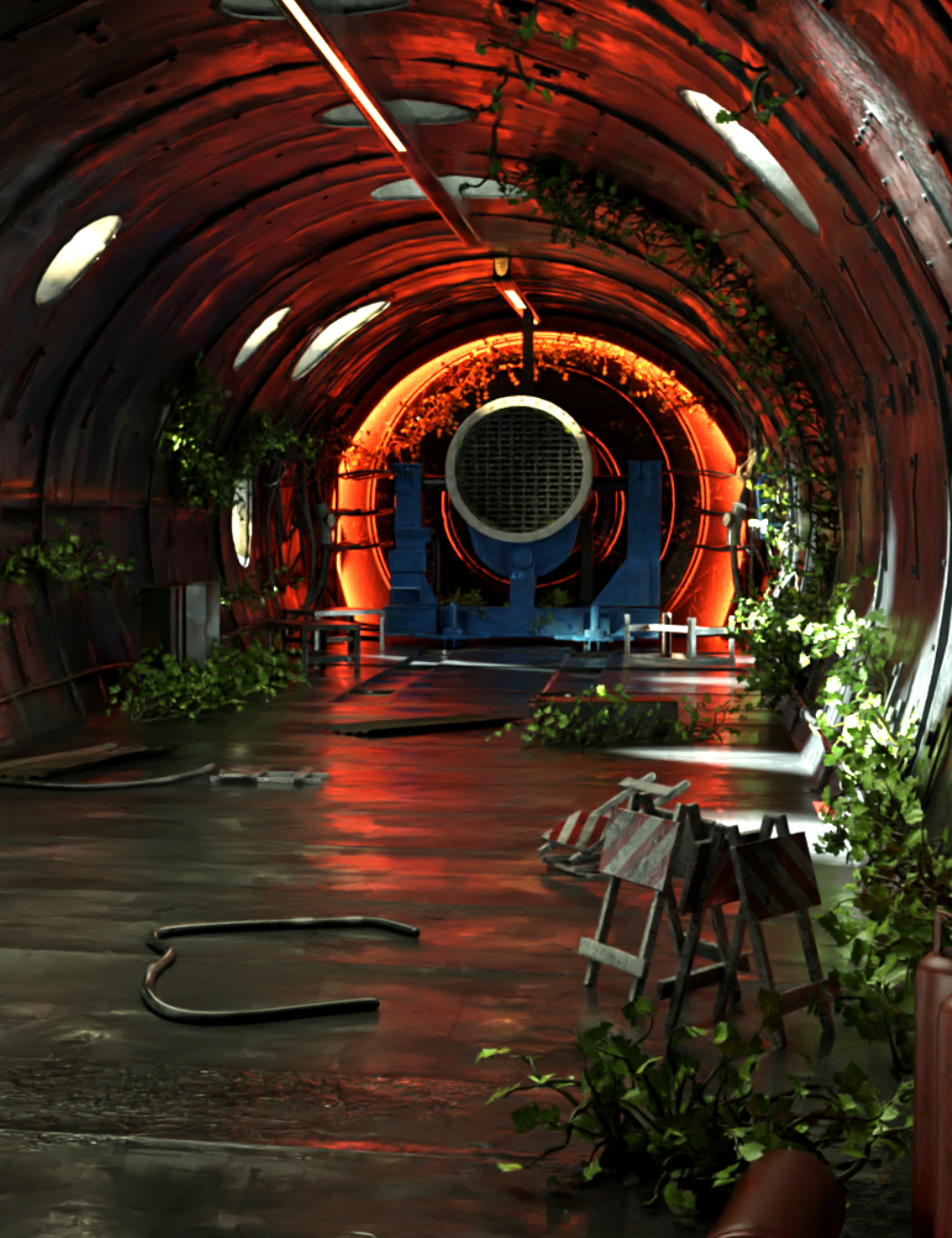The photograph depicts the interior of a rounded tunnel or tube, measuring approximately six inches high and five inches wide. The bottom half of the image highlights clean, shiny concrete flooring. In the lower right corner, green vines extend from the floor and climb up the side of the tunnel, accompanying white and red striped barrier boards. The top half showcases the tunnel’s curved ceiling adorned with round openings that allow sunlight to filter through. At the tunnel's far end, a circular vent encased in a blue metal framework is visible. The area near the vent is illuminated with an orange hue, enhancing the appearance of the green foliage. Scattered towards the sides are various plants, including vines that hang from the ceiling. The tunnel, possibly repurposed as a living space or passageway, also contains some wooden items on the floor and easel signs indicating caution or work ahead.